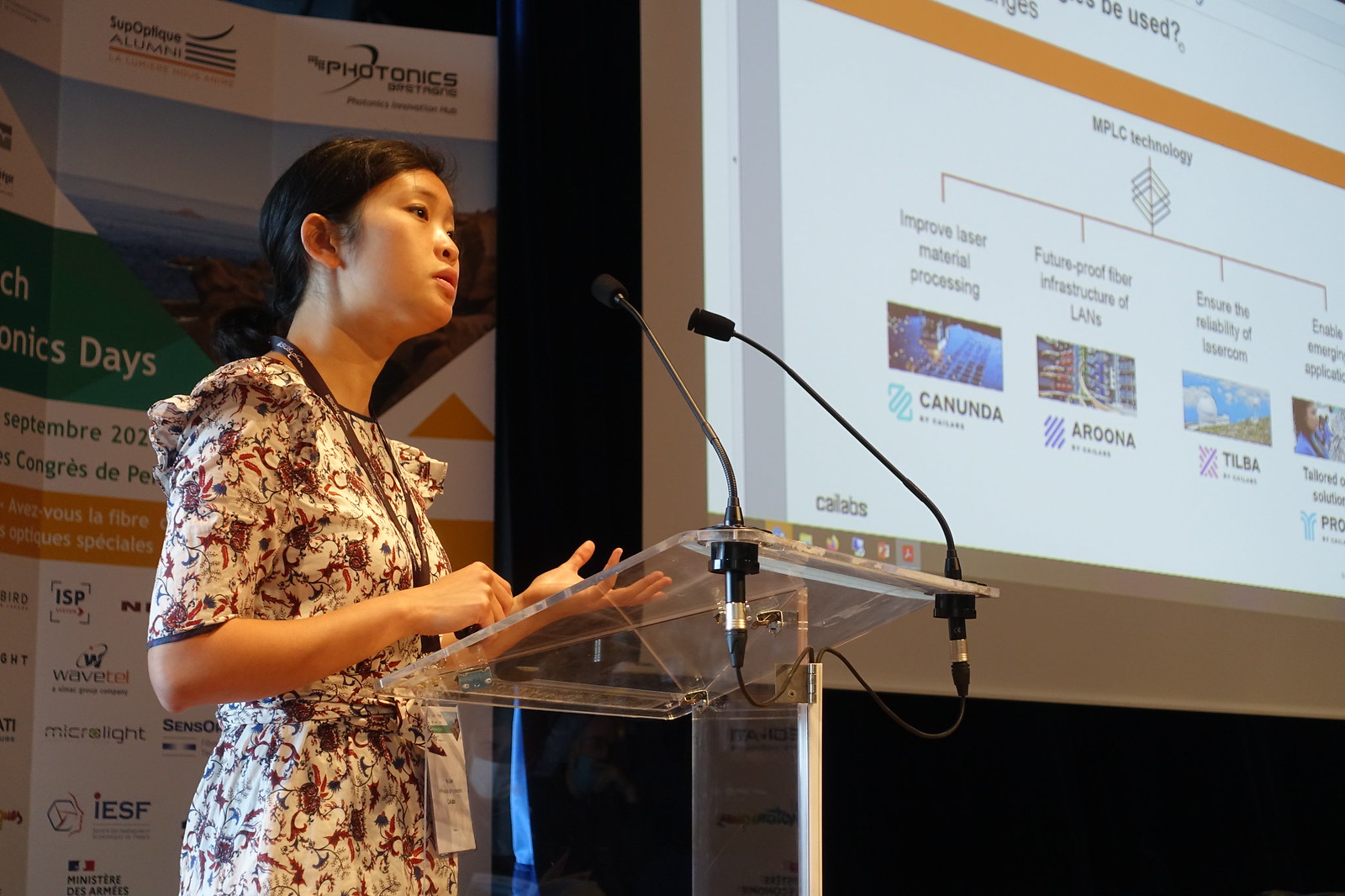In this detailed image, an Asian woman with short hair is standing centered behind a glass-topped podium, speaking into two black microphones. She is wearing a patterned dress predominantly featuring colors like white, blue, purple, and maroon, and has a lanyard around her neck. She uses her hands expressively; her left hand is gesturing, while her right hand rests on the podium. The setting appears to be an indoor presentation or conference.

Behind her, there are multiple signs and banners. One prominent banner in the background partially displays the word "photonics" along with segments of text reading "…omics" and "… days" in white letters on a green background. There is also a tall, detailed sign to her left featuring schematics and technology descriptions, including phrases like "MPLC technology," "improve your material processing," and "future ground infrastructure." Another visible detail includes a screen monitor on the right side of the image displaying fragments of logos and text, including "CANUNDA," "AROONA," and "TLBA," each accompanied by a corresponding image.

The variety of colors in the image includes white, black, gray, orange, blue, purple, light blue, maroon, and green. Despite the clarity of some elements, parts of the text and images are cut off or difficult to read, giving an incomplete view of the background materials. The overall scene indicates the woman is addressing an audience, likely as part of a formal event or presentation.